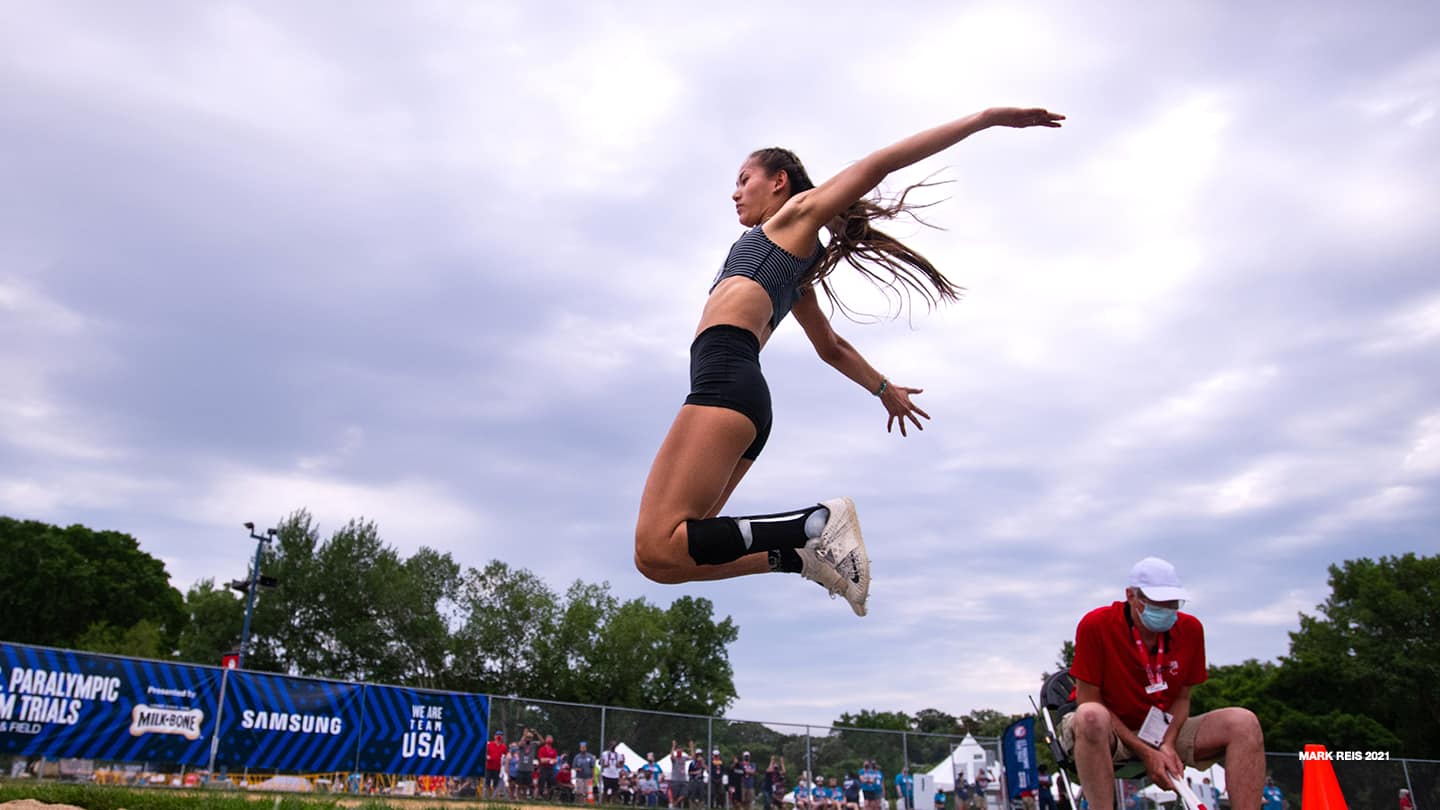This captivating image captures the intensity of a woman athlete mid-leap during a track and field event. Suspended in the air, her body is composed in an aerodynamic form; her knees are bent with legs curved behind her, arms are stretched out in a V behind her back, and her brown hair trails gracefully. She is dressed in a gray sports bra, black biker shorts, and white shoes, with one foot adorned in either a brace or a long black sock. Below her, a man dressed in a red short-sleeved polo shirt, khaki shorts, white baseball cap, and blue COVID mask, sits on a chair, looking down. An orange cone is positioned next to him. The background is bustling with a crowd behind a chain-link fence, intently observing the event. Advertisements for the Paralympic Trials, sponsored by Samsung, Milk-Bone, and Team USA, are prominently displayed on banners affixed to the fence. Above the scene, a dreamy blue sky with clouds completes this vivid capture of athletic prowess and the event's vibrant atmosphere.